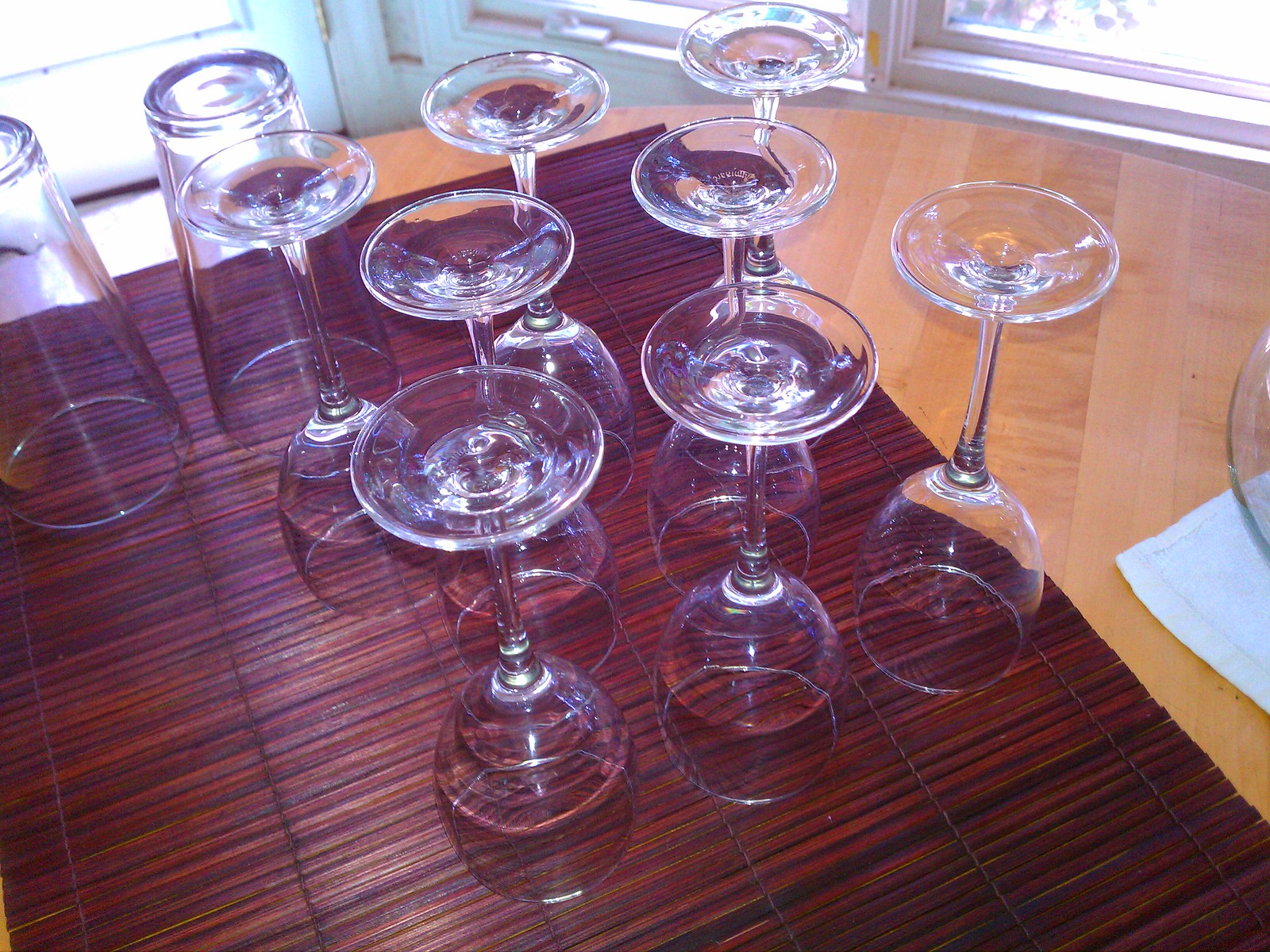This photograph depicts an orderly arrangement of clear glasses turned upside down for drying. Centered on a rolled-out dark brown, rattan-type mat, the display includes eight wine glasses and two Pilsner glasses, all transparent and positioned neatly. The mat rests on a light brown, wooden table, adding a rustic charm to the scene. In the background, windows bordered in white allow sunlight to stream in, enhancing the serene ambiance. Additionally, a white towel is visible to the left, holding an indistinguishable glass object. The composition is free of any text, focusing solely on the juxtaposition of the glasses against their natural wooden backdrop.